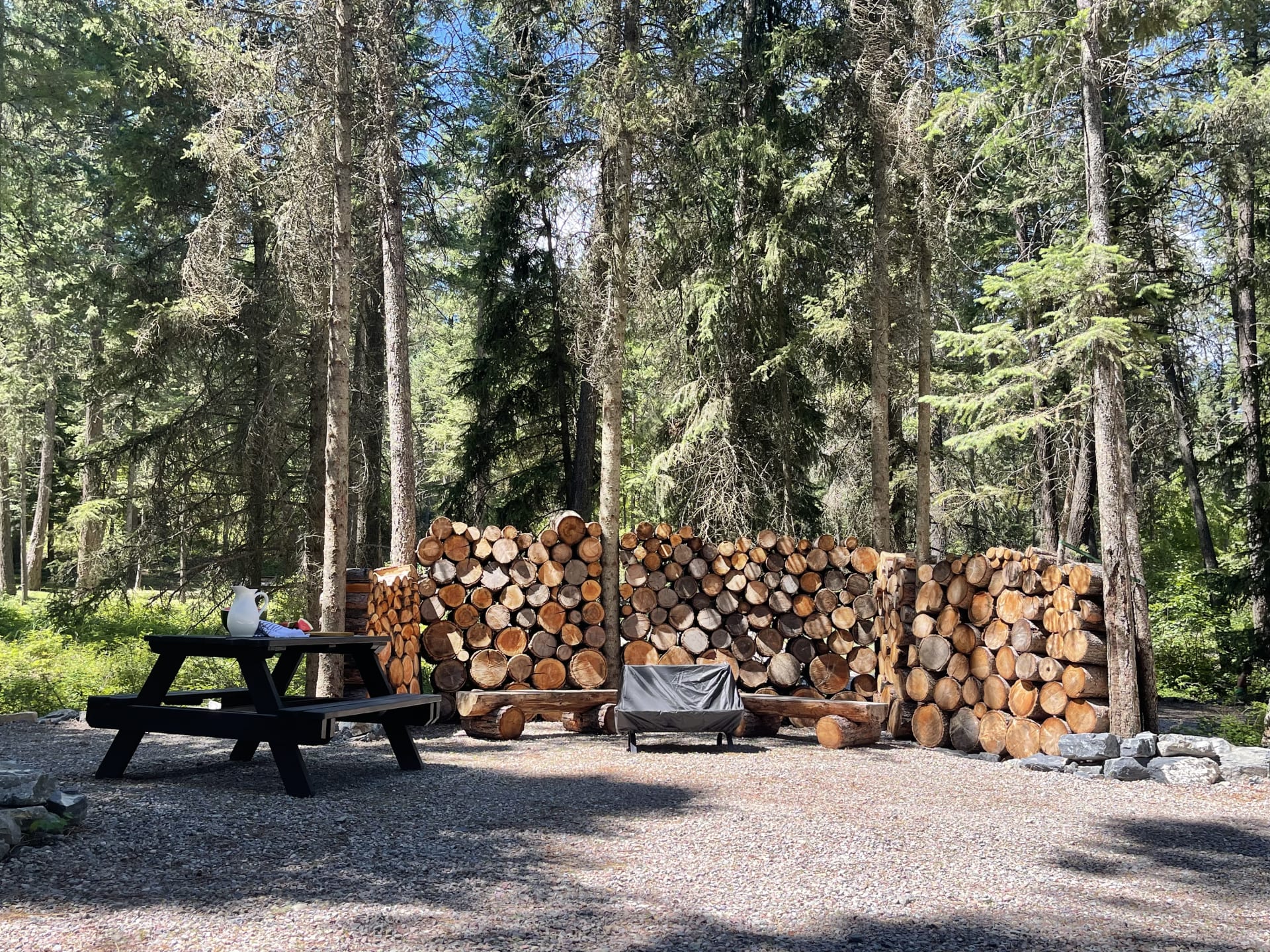The photograph captures a serene outdoor campsite set against a backdrop of tall, slender pine and evergreen trees reaching up to a bright blue, nearly cloudless sky. The campsite itself features a gravel and dirt ground with the sun casting shadows from the trees above. Central to the foreground, there is a black wooden picnic table adorned with a distinct white pitcher and various other objects. Encircling the area in a semi-circle are neatly stacked logs of firewood, organized between the tree trunks. In front of this log wall are two rustic benches, crafted simply from cut logs. Additionally, a feature resembling either a covered grill or a bench stands prominently within the camp's log perimeter. Large gray stones form a fire circle, partially visible to the left edge of the image. The overall ambiance suggests a peaceful, well-organized camping spot amidst a dense and tranquil forest.